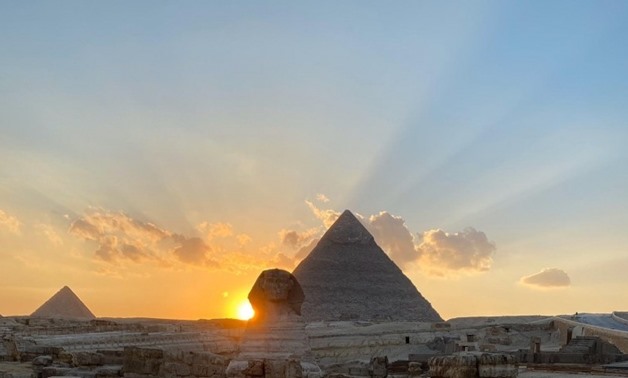This captivating photograph captures the sun peeking over the horizon, either at dawn or sunset, at the iconic Great Pyramids of Egypt. Dominating the foreground is the majestic Sphinx, gazing directly at the viewer while also glancing toward the edge of the nearest pyramid. Despite its weathered appearance and missing nose, the Sphinx retains its ancient splendor, showcasing the effects of millennia of wind and sun erosion. Behind it stand two pyramids, the larger of which juts prominently into the sky, while the smaller one sits slightly to the left. The sky above transitions from a morning glow of orange and pink near the horizon to a striking blue, punctuated by clouds through which sunlight streams dramatically. Together, these elements create a powerful and timeless tableau that evokes the grandeur of ancient Egypt.